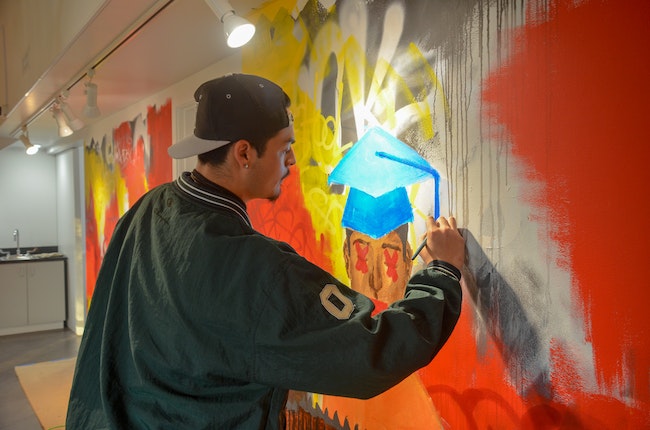The photograph captures a male artist in the midst of painting a mural on an orange and yellow wall, inside a room seemingly set up for mural creation. The artist, seen from his right side, wears a black long-sleeve baseball jacket emblazoned with a white zero above his elbow, a black and gray baseball cap worn backwards, and a right earring. He sports a goatee and mustache. The mural features a graduation scene, with a figure in a cap and gown; the tassel of the blue cap is currently being painted by the artist, who holds a paintbrush in his right hand. Notably, the figure in the mural has two red Xs over their eyes, adding a striking detail to the painting. Overhead, several white lights on a rail illuminate the workspace, and a sink with a faucet is visible in the far left background of the room. The wall is vibrant with varying colors, including red, blue, yellow, and white, enhancing the dynamic and creative atmosphere of the scene.